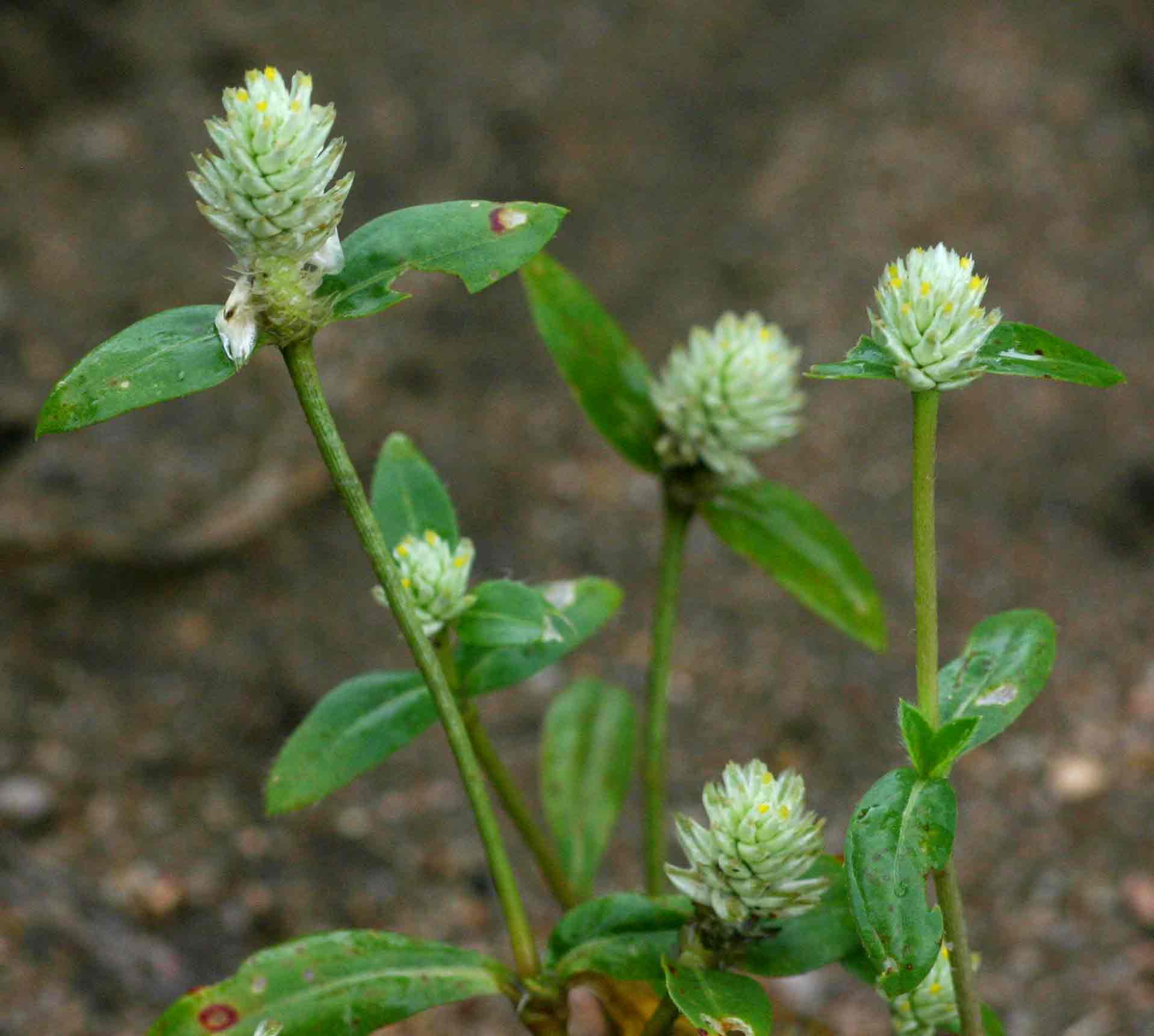The image features a cluster of five flowers with long stalks and medium-sized leaves, set against a brownish-black dirt surface with exposed tree roots. The flowers resemble pine cones, with buds in a light green hue transitioning to pale yellow at the tips. The arrangement includes three flowers at the top, two in the middle, and one near the bottom of the image. The leaves are bright green, some of which exhibit bite marks or red blemishes, suggesting insect activity or possible disease.